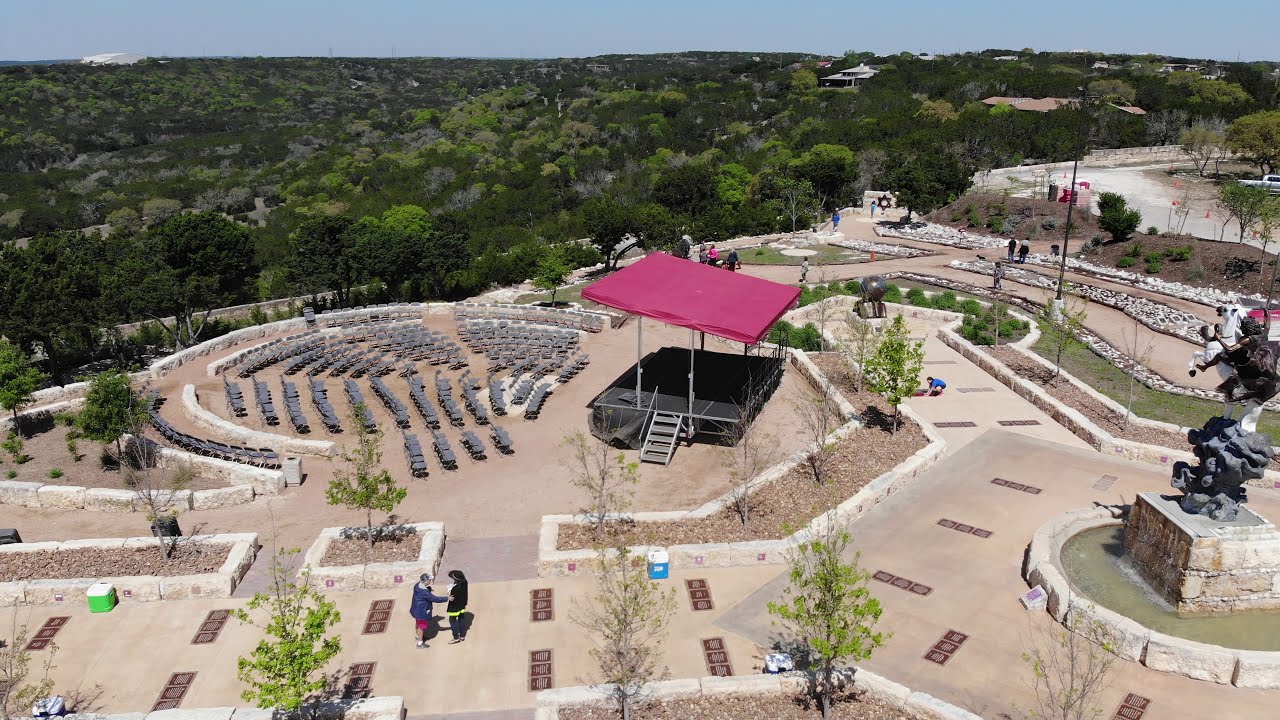This aerial photograph captures a spacious outdoor venue set up for an upcoming event, possibly a concert or show. Central to the image is a black stage with a red canopy top, accessible via five silver stairs. Surrounding the stage is a circular arrangement of gray seats, currently unoccupied, bordered by a stone walkway. 

On the walkway, two individuals can be seen facing each other; one extends an arm as if in greeting or direction. These two people are distinct, with one wearing a blue hoodie and red shorts and the other in a red and black hoodie with dark pants. Nearby, a green cooler with a white top and a blue cooler with a white top are present, along with another person in a blue shirt. 

Further elements of interest include various stone flower beds bordering the walkway, filled with green foliage and punctuated by brown mulch. A striking statue of a white horse with a black knight stands prominently, its base composed of tan and black stone. This venue is set in a clearing, surrounded by lush greenery and trees. In the top right corner of the photo, a body of greenish water is visible, with additional figures walking in the distance. The setting includes outdoor lighting fixtures in tan and black colors, adding to the preparation for the forthcoming event.